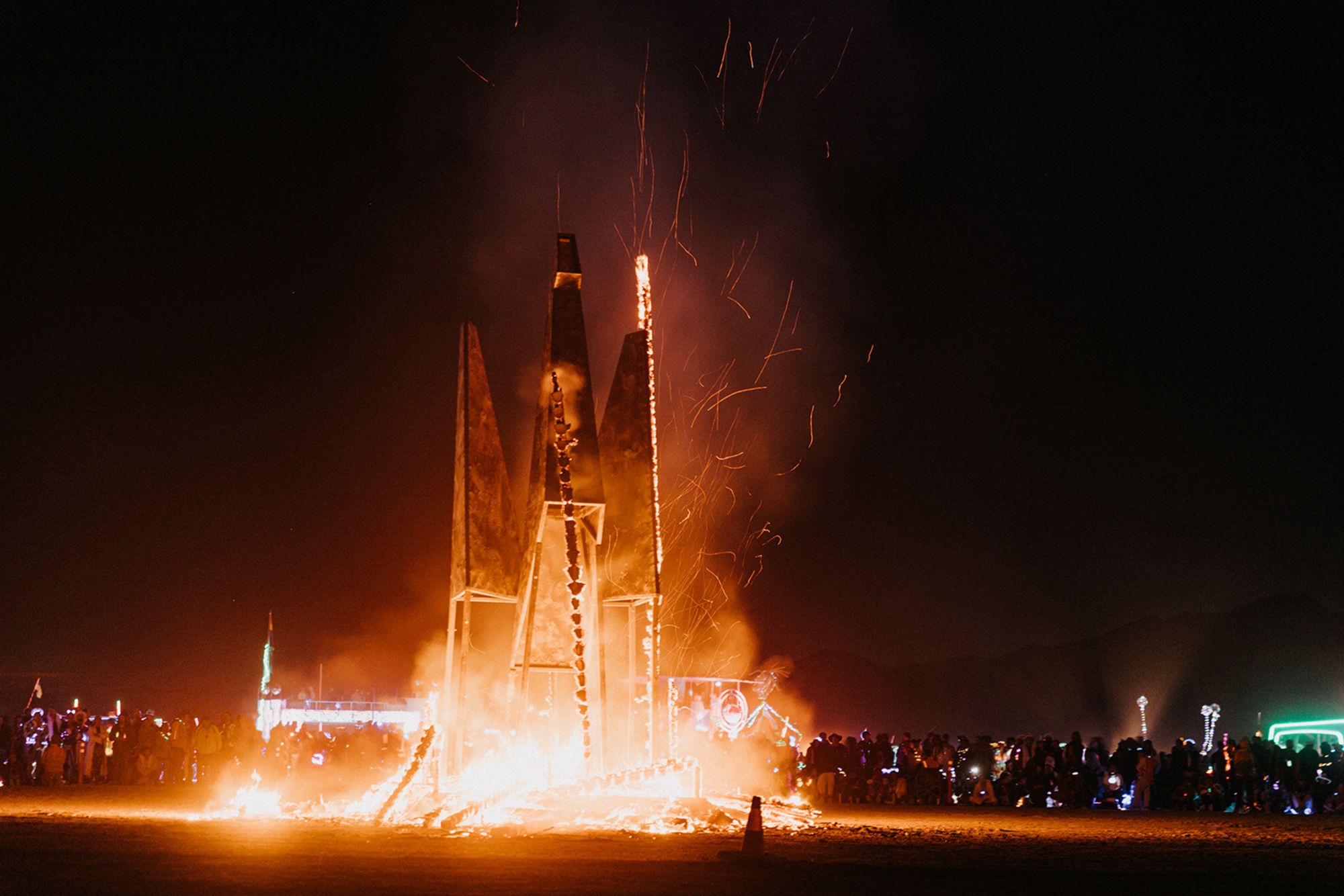The nighttime image taken at the Burning Man Festival captures a dramatic scene dominated by a wooden or possibly mixed-material art installation, which is being engulfed in flames. The sky is pitch black, adding to the intensity of the scene. The installation, resembling a triangular, castle-like tower with three pinnacles—the middle being the tallest—is catching fire from its base, which glows a fierce red and orange. The structure itself appears to have some sort of canvas covering over the triangular sections, contributing to the flames. Around the fiery tower, a large crowd of people is gathered, their appearances obscure except for the neon lights adorning their heads and costumes. To the right of the flaming structure, a safety cone silhouette is visible on the ground. The ground itself is leveled dirt, further emphasizing the stark contrast and the communal nature of this bonfire event—the perfect embodiment of the Burning Man Festival's spirit.